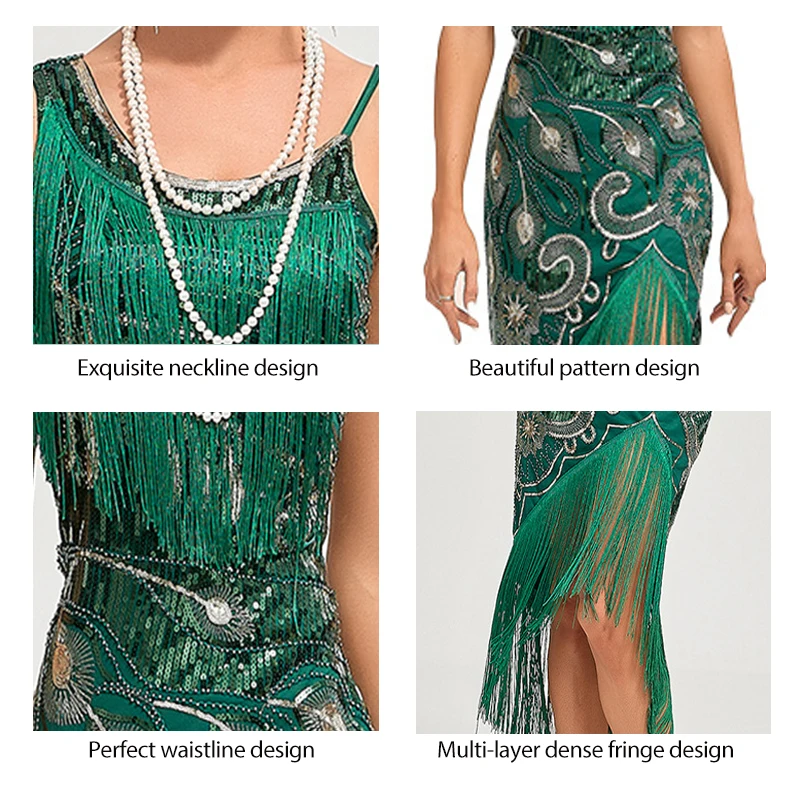This marketing-style 4-up quad photograph showcases various intricate details of a visually striking, teal-green flapper dress, reminiscent of 1920s fashion with a modern twist. The image is organized into a grid of four perfectly square, uniformly sized photos against a white background, each highlighting different parts of the dress on a light-skinned model, whose face is not visible.

In the top left photo, the exquisite neckline of the dress features a heavy band of teal-green fringe cascading from a black beaded neckline. The model accessorizes with a double string of white pearls. The text below this section reads, "Exquisite Neckline Design."

The top right photo displays the dress’s beautiful pattern design from just below the bust to above the knees. The heavily embroidered and beaded fabric, featuring peacock feather-inspired designs in bright teal and black, covers the lower torso and hips. A notable upside-down V cutout on the left thigh accentuates the intricate appliques and is adorned with a band of fringe.

The bottom left photo focuses on the perfect waistline design, showing the dress from the chest down to the waist. Here, green fringe and sequins contrast against a black background with elaborate beading and embroidery that include silver sequins or piping.

The bottom right photo showcases the multi-layer dense fringe design of the skirt from just below the hips to above the ankles. The dress fits snugly over the hips and flares out with long 12-inch teal-green fringe, enhancing its movement. This section also emphasizes the asymmetrical cut and the dynamic nature of the flowing fringe.

Collectively, the images provide a detailed view of the dress’s intricate, flapper-era inspired design, emphasizing its modern elegance through exquisite detail and craftsmanship.